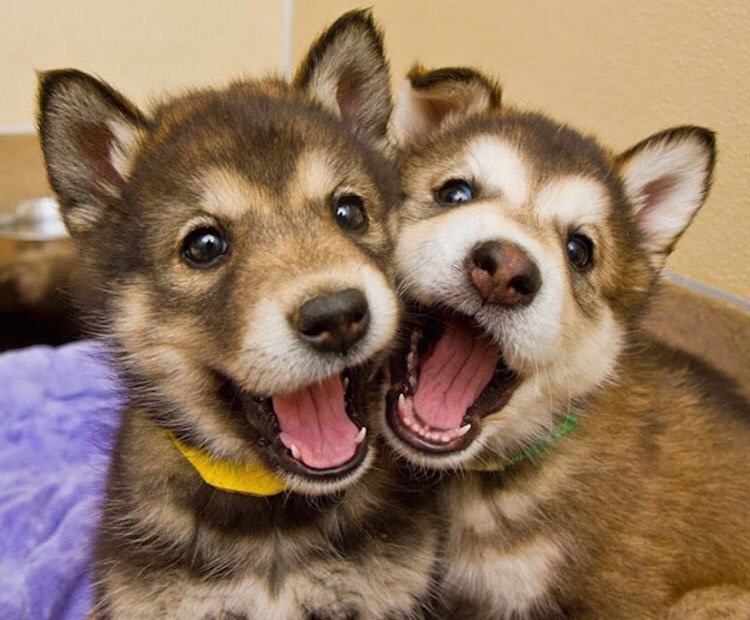This indoor photograph captures two adorable husky puppies sitting on a purple blanket that might be a bed. The tan walls in the background frame their playful interaction. Both puppies have their mouths open, revealing their puppy teeth, and their heads are pressed together in what looks to be a moment of mid-play. Their fur is a mix of brown and white, with the puppy on the left sporting orange accents around its face and a yellow bandana around its neck. The right puppy has more white around its eyes and mouth, and its green collar is partially tucked in. Their ears are pointy, but one of the right puppy's ears is drooping slightly. Both puppies have brown eyes and appear to be under eight weeks old, capturing a snapshot of youthful joy and sibling bonding.